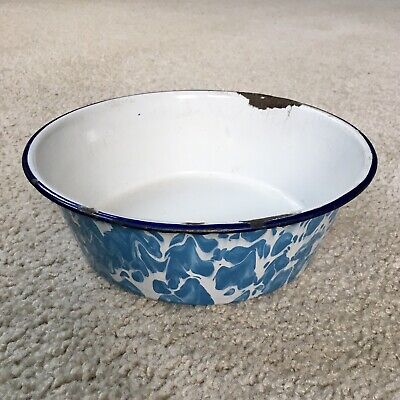The photograph captures a close-up image of a ceramic or porcelain pet bowl, likely intended for a dog or cat. The bowl, prominently positioned in the frame, rests on a clean, beige carpet, suggesting an indoor setting. The bowl features a white interior and a black outer rim, with a noticeable chip on the top inside edge that exposes black underneath. The exterior boasts a striking blue and white marbled pattern, reminiscent of abstract waves or a school of fish swimming through the design. The bowl is relatively shallow, standing only a few inches high, but its wide opening is accentuated by a flared lip. The detailed craftsmanship includes a pewter-colored, ribbed edging around the rim, adding a touch of elegance to the overall design. Despite a small area of rust or worn enameling, the bowl remains a visually appealing piece that stands out against the neutral carpet backdrop.